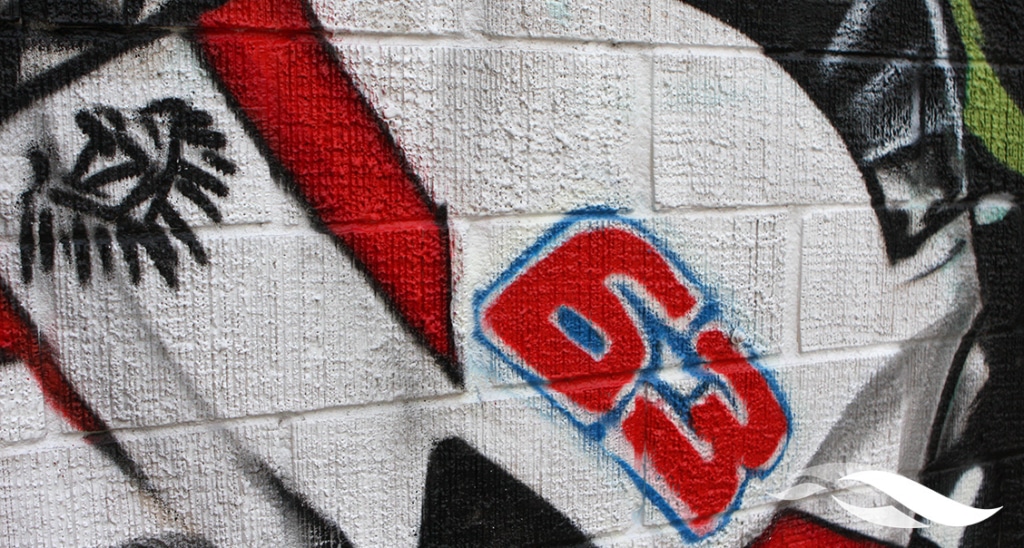A detailed graffiti mural is depicted on a mostly white concrete wall. The focal point is the number "63" painted in bold red block numbers with a blue outline, positioned in the middle of the image. Above the number, a red line, which resembles a ribbon and is outlined in black, descends from the top left corner. This ribbon cuts diagonally through the center of the mural. To the right of the number, the wall features intricate designs with a mix of black, yellow, and green details, giving an abstract impression that might be taken as a bird or a piece of sports equipment, like a hockey jersey or helmet. Below the "63," touches of red and black paint are scattered, suggesting dynamic, spray-painted embellishments. The mural includes a variety of interconnected abstract patterns and symbols, adding depth and complexity to the artwork. In the lower right corner, a small white watermark resembling two cresting waves can be seen, contributing a subtle signature to the otherwise vibrant graffiti scene.